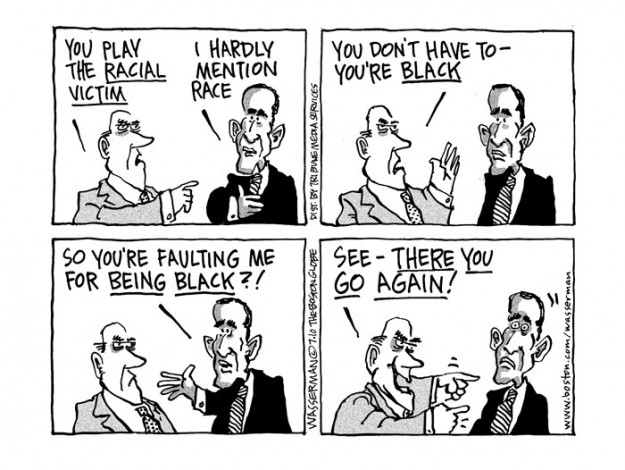In this black and white political cartoon, illustrated in four panels, a white man in a suit engages in a charged conversation with a black man, who appears to be a caricature of Barack Obama. The dialogue begins with the white man accusing the black man of playing the "racial victim." Obama retorts by saying, "I hardly mention race." The white man counters, "You don't have to, you're black," to which Obama responds, "So you're faulting me for being black?" The white man concludes with, "See, there you go again," leaving Obama looking dumbfounded. The simplistic monochrome palette of black, white, and gray highlights the starkness of their interaction, which critiques societal racial dialogues. The illustration is signed by Wasserman, suggesting a known liberal commentator behind this provocative piece.